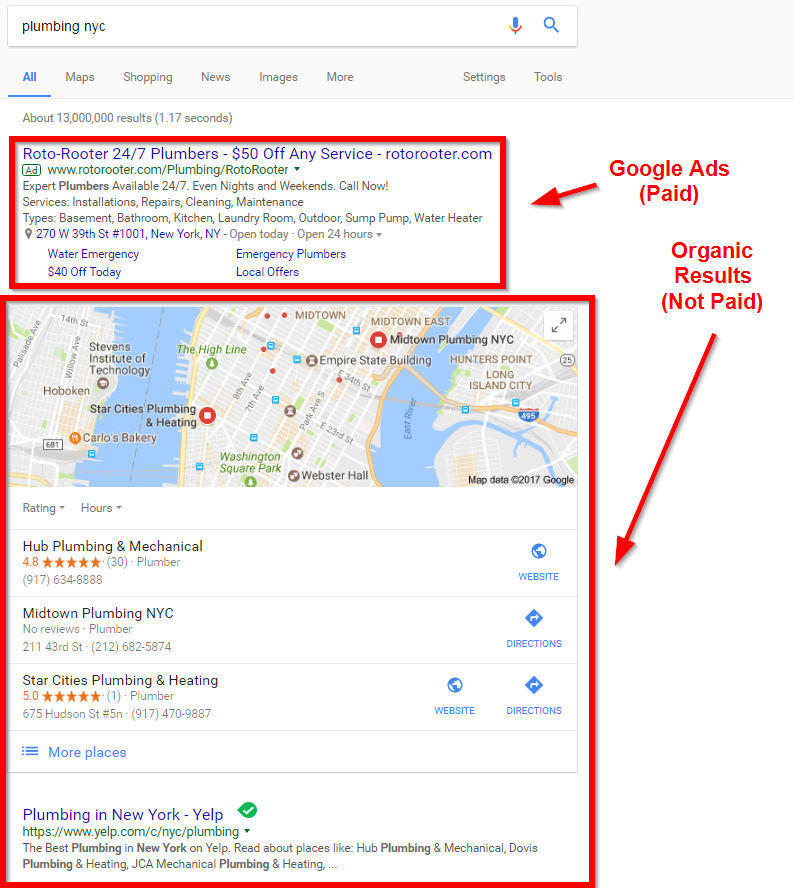The screenshot displays a search results page for the query "plumbing NYC." At the top, a search box contains the typed text "plumbing NYC" against a light gray banner. Below the banner, various dropdown topics are available, including "All," "Maps," "Shopping," "News," "Images," "More," "Settings," and "Tools," with "All" being underlined.

Just beneath these dropdown options, the text indicates there are "About 13 million results." Dominating the upper part of the search results is a section enclosed within a thick red outline, labeled as "Google Ads - Paid." A red arrow on the right column points to this area, identifying it as a section for paid advertisements. The highlighted ad is for "Roto-Rooter," offering 24/7 plumbing services with a "$50 off any service" deal, and includes a link to rotorooter.com.

The lower section of the search results contains another arrow, labeled "Organic Results (Not Paid)." This section, free from paid advertisements, shows the standard results generated by the search engine algorithm. The top part of this section features a map displaying three listings for plumbing companies: Hub Plumbing and Mechanical, Midtown Plumbing NYC, and Star Cities Plumbing and Heating. Additionally, at the bottom of this section, there is a link to "Plumbing in New York - Yelp."

The overall image lacks borders on the left, right, and bottom sides, presenting a clean snapshot of a search results page with both paid and organic listings for plumbing services in New York City.